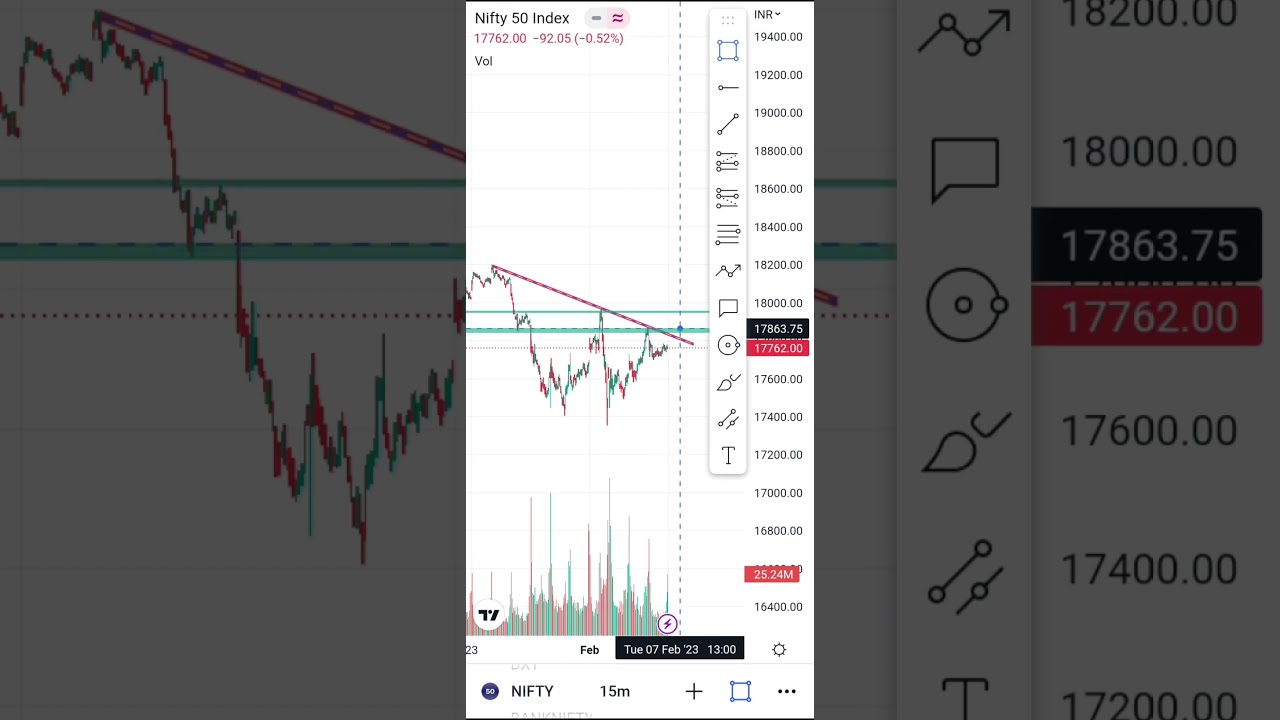The image is a detailed screenshot of a financial utility displaying the trading performance of the Nifty Fifty Index. The central panel showcases a detailed candlestick graph, capturing the stock's fluctuation with precise increments. The graph’s colors, red and green, denote downward and upward value changes respectively, with a corresponding bar graph along the bottom for volume. The Nifty Fifty Index closed at 17,762.00, marking a decline of 92.05 points or -0.52%. Highlighted numbers in the background ($17,863.75 and $17,762.00) appear to be integral to the calculations presented. The date at the bottom reads Tuesday, 7 Feb, 23 at 13:00. The right section features close-up tools and instruments, suggesting the image might have been captured during the graph's creation. The graph’s Y-axis ranges from $19,400 at the top to $16,400 at the bottom. Additionally, a currency dropdown menu on the top right indicates INR. The chart's annotations include a summary of 15-minute increments displaying daily trading volumes, further detailed with high-low markers of the year's performance, reflecting the asset’s oscillation between its highest and lowest trading points.